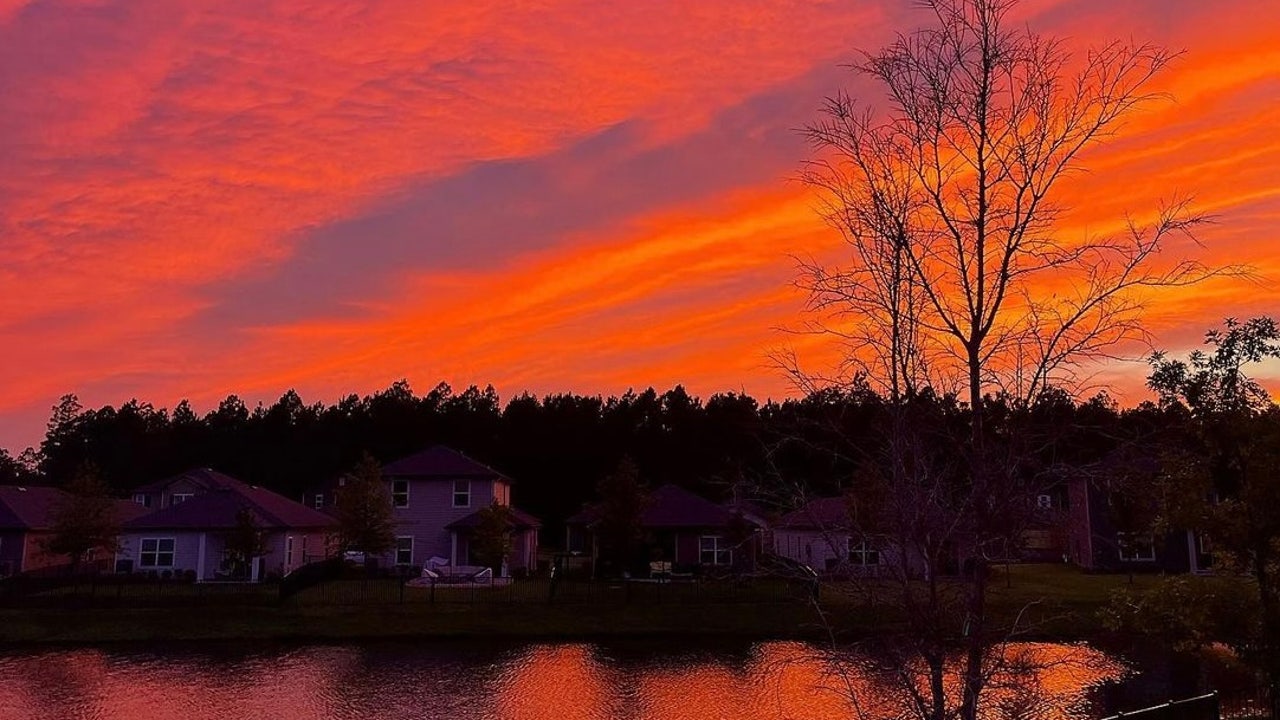The image captures a serene, moody sunset over a neighborhood block set against a backdrop of a dense tree line and calm body of water, likely a lake, reflecting the vibrant colors of the sky. The sunset dominates, casting brilliant orange hues with accents of yellow, pink, and traces of purple, creating an almost ethereal glow that illuminates the scene. The sky features wispy cirrus clouds and patches of light blue and white amidst the orange tint. Below the sky, a row of suburban houses, varying in height and size, stands silhouetted against the light. Some houses are two-story, others are single-story, with white tan exteriors and dark, pointed roofs. In front of the houses stretches a grassy area leading to the water's edge, where the smooth surface of the lake mirrors the sunset’s fiery tones. The foreground and side of the image feature trees, some bearing green leaves and others starkly bare, their leafless branches etched darkly against the colorful sky, enhancing the autumn or winter atmosphere. The overall composition, with its horizontal crop and balance of shadow and light, exudes a rich contrast between the vibrant sunset and the silhouetted landscape, bringing a tranquil yet dramatic feel to the photo.